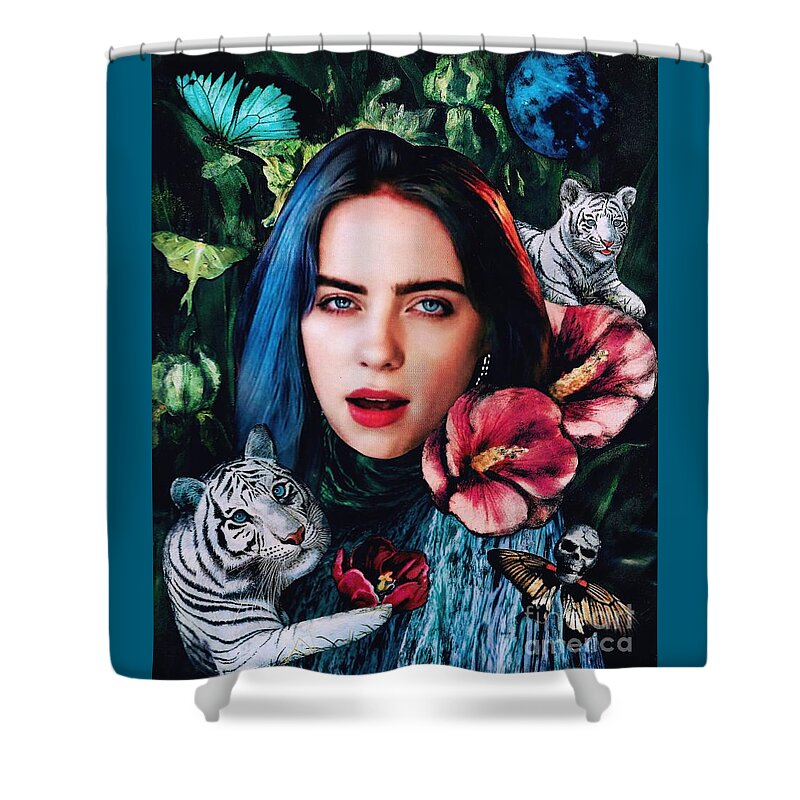The image showcases a vivid and surreal artwork, possibly on a shower curtain or velvet poster, featuring a striking woman with distinctly colored hair: long black locks highlighted with purplish and orange-reddish streaks. Her lifelike facial features include thick eyebrows, blue eyes, and pinkish-red lipstick. Surrounding the woman are two majestic white and black striped tigers with piercing blue eyes; one positioned near her jawline and the other above and behind her. Enveloping the scene are various elements, adding to its eerie and captivating allure. Pinkish-white flowers surround her head, while butterflies, some with skull motifs, flutter nearby. The moon, painted in blue hues, glows in the backdrop against the predominantly black background adorned with dark blue trimmings and aqua green accents. Additionally, a graphic indicating "Fine Art America" is subtly included at the bottom of the image. The entire composition creates an odd yet mesmerizing visual experience, blending natural and fantastical elements seamlessly.